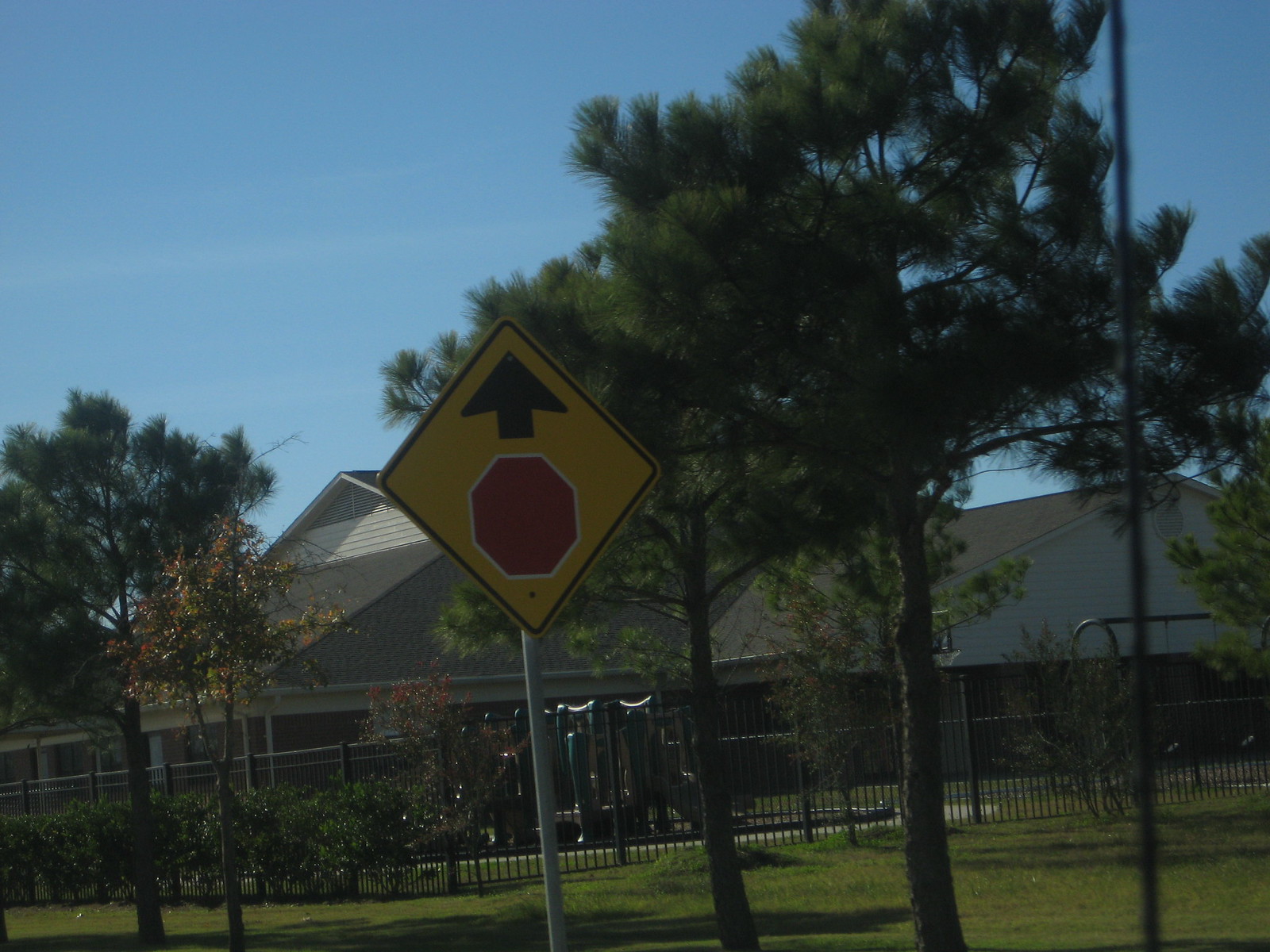This outdoor daytime photograph features a vivid blue sky occupying the upper half of the frame, contrasting with the darker, shaded lower portion of the image. Dominating the foreground are lush, green evergreen trees that stretch across the scene. Prominently placed in the lower middle of the image is a yellow diamond-shaped sign, positioned at an angle, warning of a stop sign ahead. Behind the trees, a building is partially visible, though obscured by foliage and lacking in detailed features. An iron fence can be seen running in front of the building, partially enclosing what appears to be a small playground area.